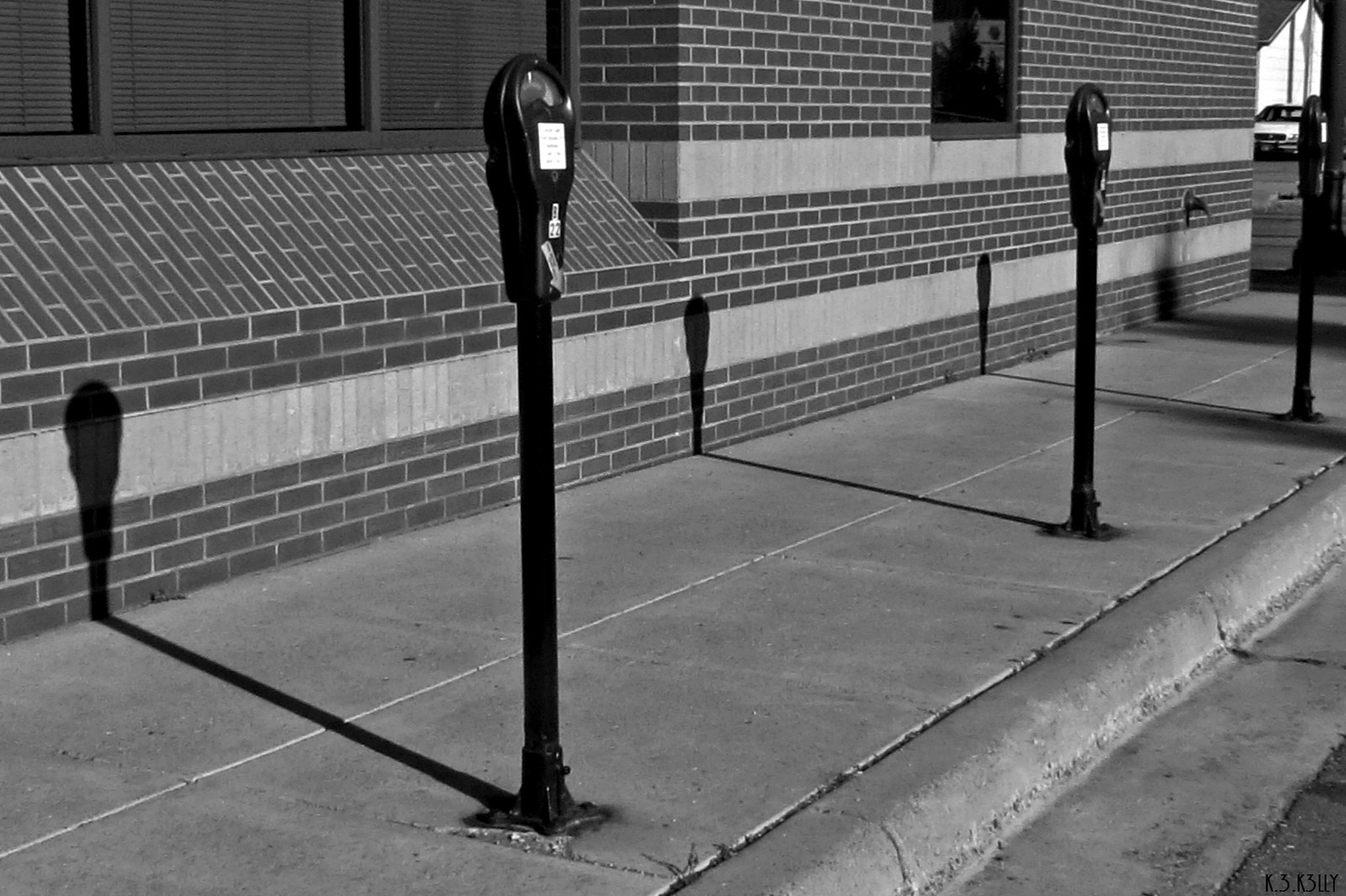In this black-and-white daylight photograph, a cityscape unfolds featuring a diagonally extending sidewalk that begins from the bottom left corner and stretches to the upper right. Centered prominently along the sidewalk are three tall, black parking meters, each adorned with a small, white information square. These meters are evenly spaced along the curb, which borders a section of the visible street in the lower right corner. The sidewalk itself comprises concrete slabs and runs adjacent to a brick building, which is visible on the left side of the image. The building's façade is detailed with dark bricks interspersed by decorative bands of white bricks, and three windows are visible in the upper left part of the image. The sun casts long shadows of the parking meters onto the sidewalk and building, adding to the sharp contrast of the image. In the upper right corner, part of a white car can be seen, its front end facing the camera. Nestling into this visual harmony is the absence of people, enhancing the timeless, serene quality of the photograph.